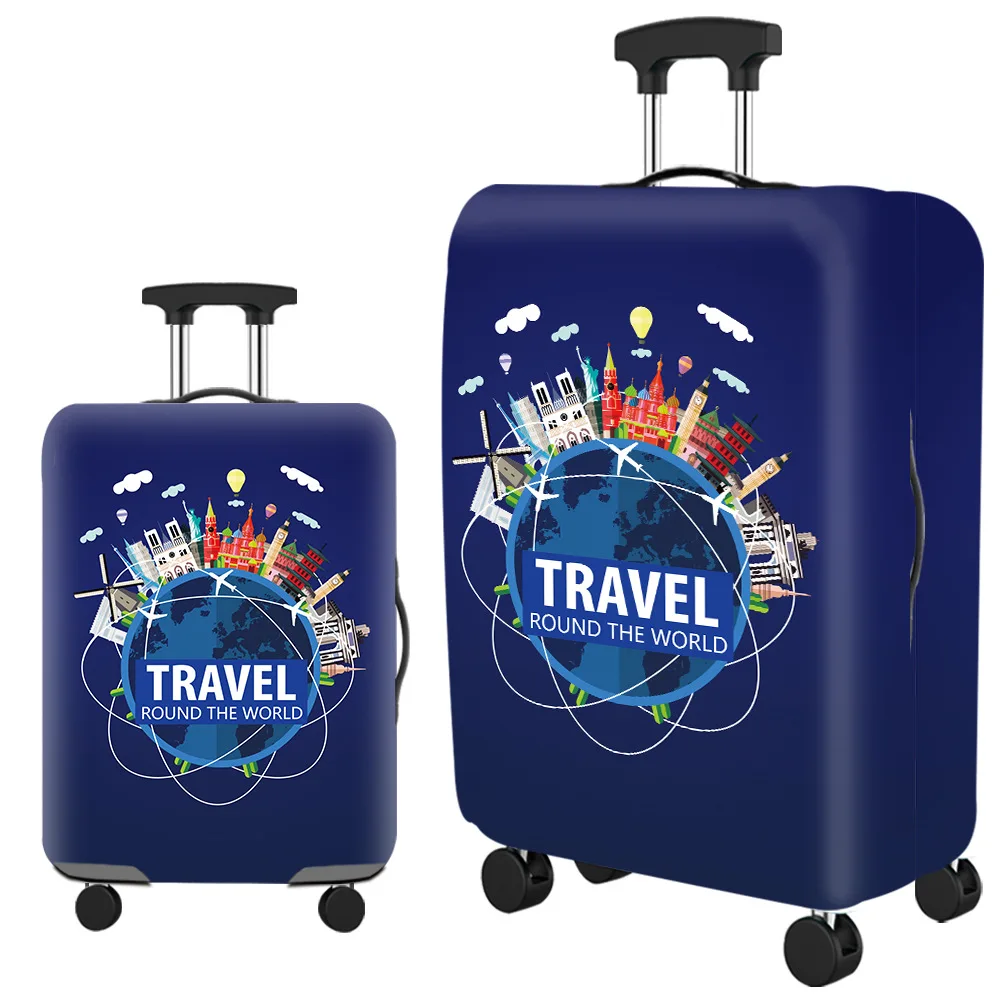This image is a detailed advertisement possibly from a shopping website showcase featuring a dark blue suitcase with a travel-themed design. The left side of the image displays a smaller suitcase head-on, emphasizing its two black wheels and extendable handle with chrome-like edges. The suitcase prominently features an illustration of a globe at the center, surrounded by cartoon buildings, airplanes, clouds, and hot air balloons, with the text “TRAVEL AROUND THE WORLD” styled in white letters on a blue background. To the right, a larger version of the same suitcase is presented at a three-quarter angle, revealing both the front and one of its sides. This larger suitcase, which is approximately one and a half times bigger, shares the same travel-centric design, including the visible small back wheels. This dual perspective highlights the suitcase's functionality and aesthetic appeal for globetrotters.